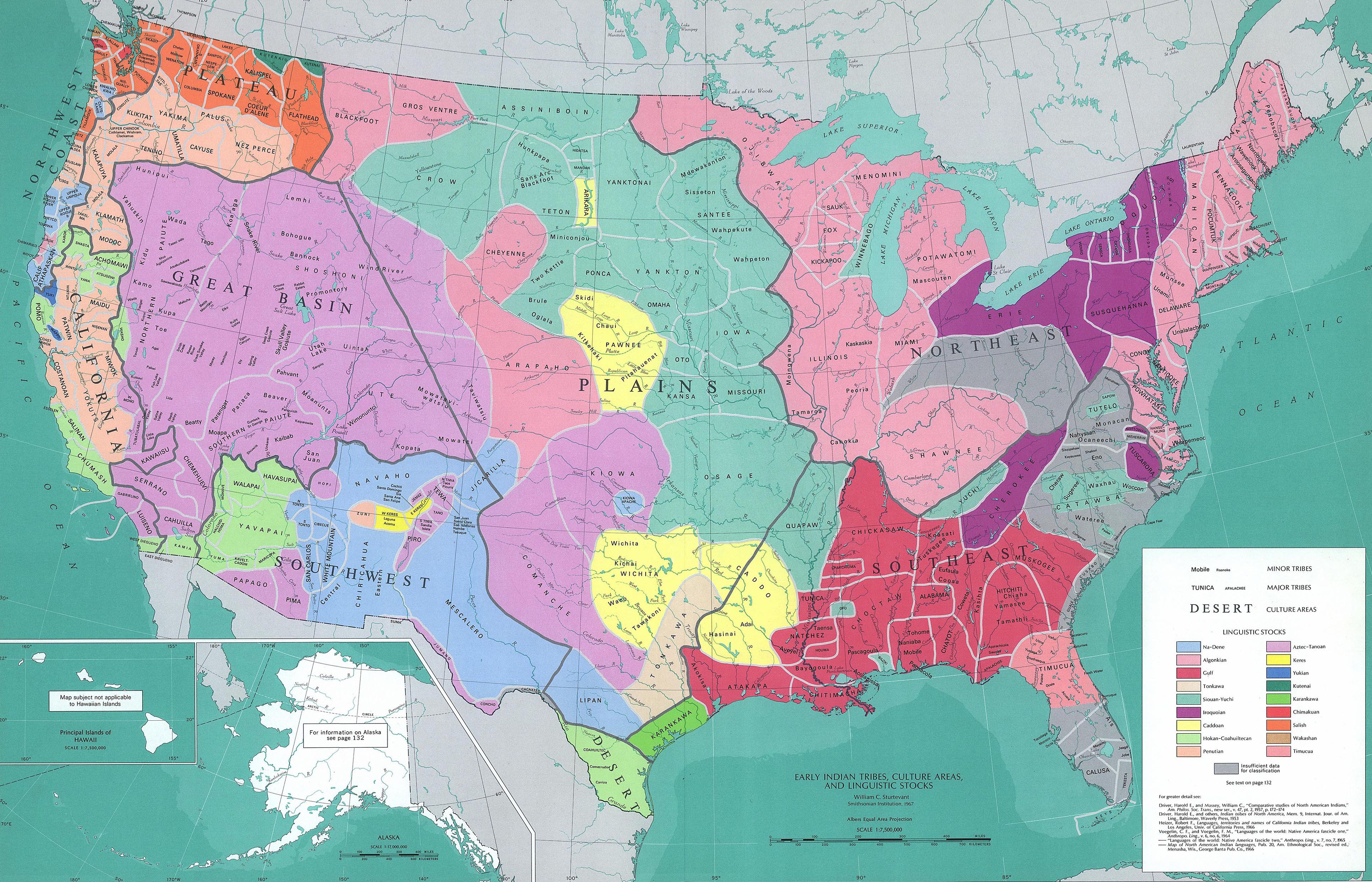A meticulously detailed color map of the United States titled "Early Indian Tribes, Culture Areas, and Linguistic Stocks" serves as the centerpiece. Although the individual states are not clearly labeled, the map provides a wealth of information through various colors indicating different linguistic stocks, as detailed in the accompanying key. The map includes a distance scale at the bottom for spatial reference. Prominent geographical features, such as the Atlantic Ocean and the Pacific Ocean, are clearly labeled, adding context to the depicted regions. An inset in the bottom left corner illustrates Alaska, expanding the map's scope. Key cultural areas such as the Great Basin, Southwest, Plains, Northeast, and California and Plateau are distinctly labeled, while Canada is represented as a gray landmass to the north. A list of sources is provided for those seeking greater detail, ensuring the map is both informative and comprehensive.